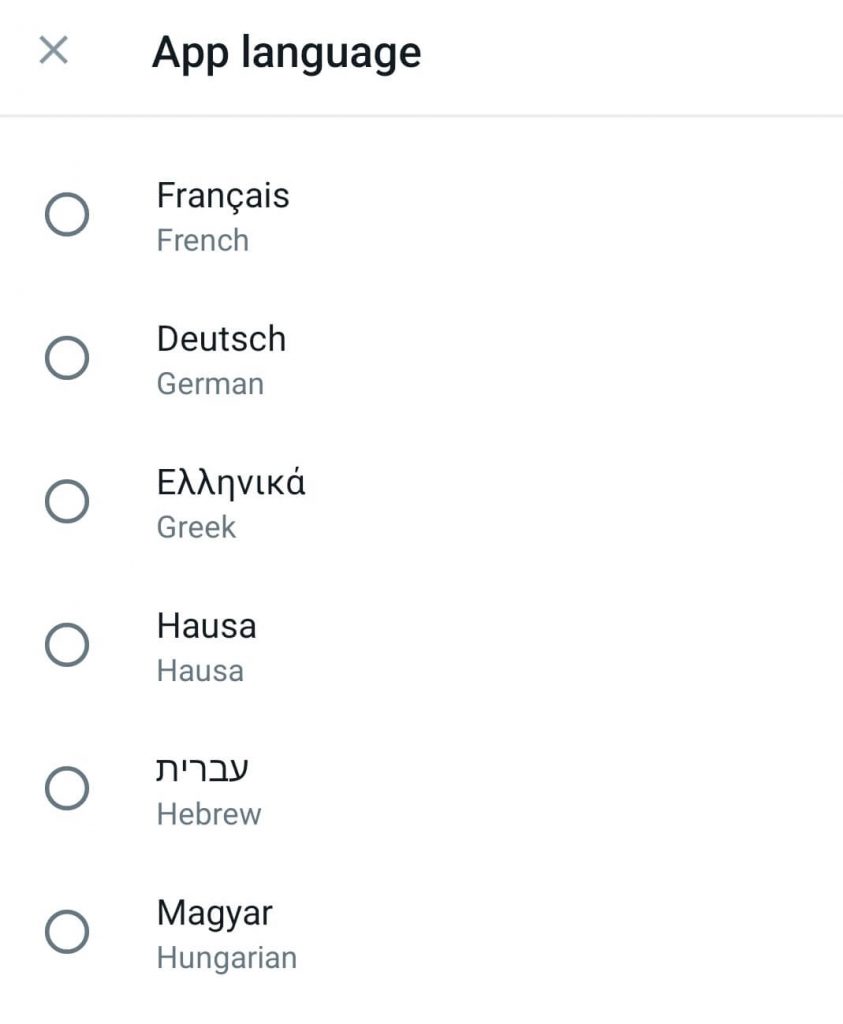Screenshot of a mobile phone interface displaying the app language settings. At the top, there is a label "App Language" with a close (X) button to the left of it. Below this, there are various selectable language options presented in individual bubbles. The available languages include French (Français), Dutch, German, Greek (Ελληνικά), Hausa, Hebrew (עברית), and Hungarian (Magyar). This screen likely allows users to choose their preferred language for the app interface, which is particularly useful for those who are traveling or for speakers of multiple languages. This feature ensures that users can interact with the app in their native or preferred language, enhancing their ability to communicate and understand the app's content, which is vital for effective use and overall user experience.